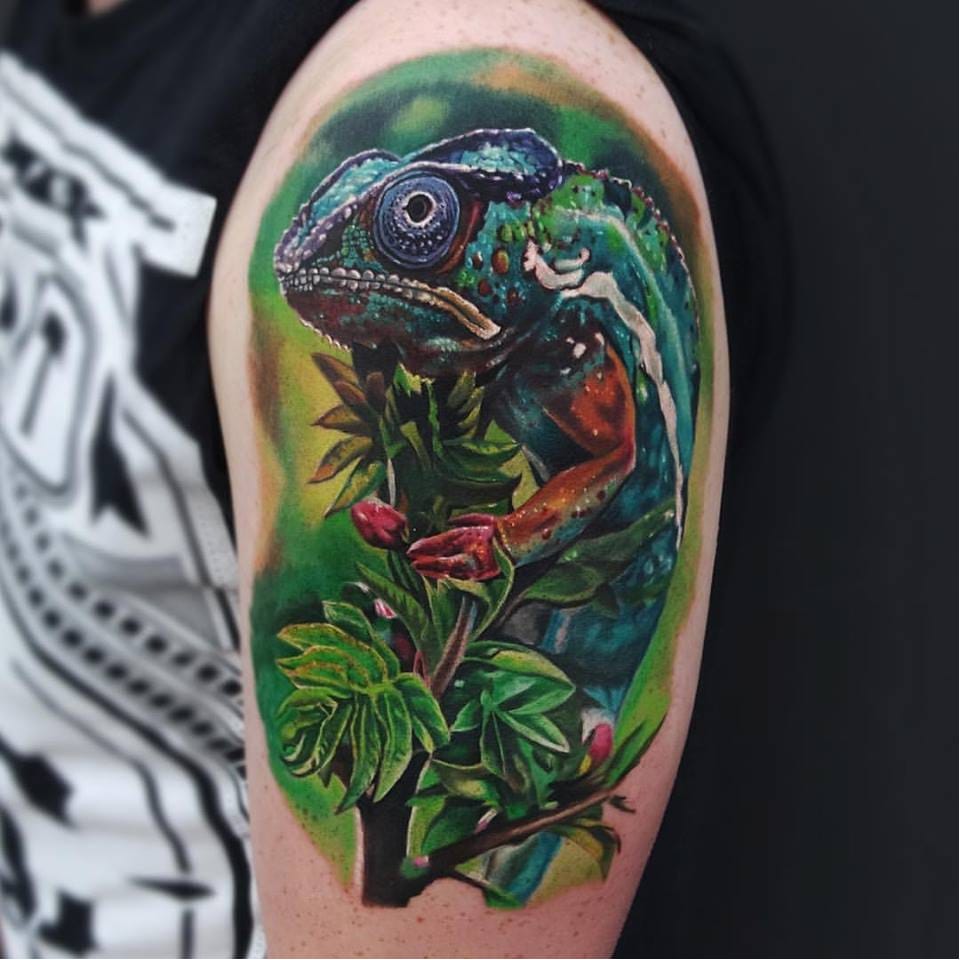The photograph depicts an intricate and colorful tattoo of a large, lifelike lizard, possibly an iguana or gecko, on a person's shoulder and extending down the side of their arm. The person wears a sleeveless black shirt that reveals their white skin. The lizard tattoo is exceptionally detailed, showcasing a vivid turquoise face, bright green and turquoise body, and reddish arms and hands. The lizard's eye is strikingly blue with a black center, while its mouth features shades of white, red, and blue. The creature is depicted crouching on a green branch adorned with small red flowers, and the branch appears quite thin, giving the impression that the lizard is crawling up it. Surrounding elements include green leaves and a brown stem, enhancing the naturalistic look of the tattoo. The overall vibrant design is accentuated further with bright green borders that frame the tattoo, making it stand out prominently against the person's skin.